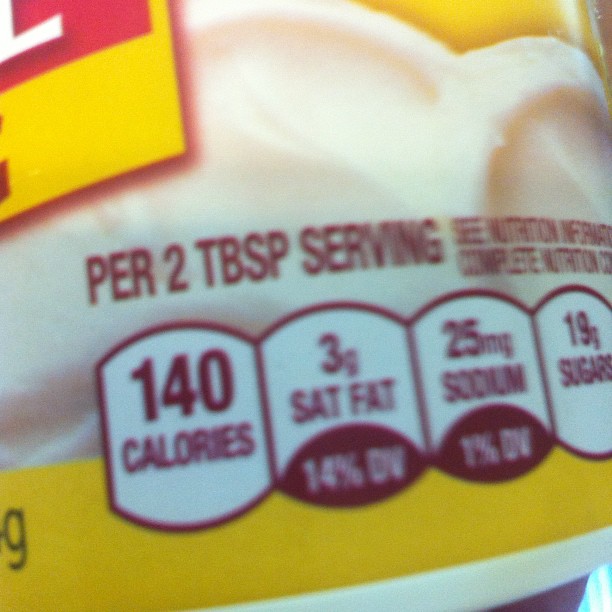This image captures a very close-up view of a yellow container, possibly holding frosting. Prominently featured in the image is the label, which is too zoomed in to clearly identify the exact product. The label has a background of yellow and depicts white frosting swirling upwards. Written in a dark burgundy or brown color, it specifies "per two tablespoons serving". To the right, though partially cut off, the label mentions "see nutritional information" followed by an incomplete "complete nutrition". Below these instructions, in a series of four oval elements, the nutritional details are displayed: 140 calories, 3 grams of saturated fat (14% Daily Value), 25 milligrams of sodium (1% Daily Value), and 19 grams of sugars. Additionally, there is a logo or label in the top left corner that is red and yellow, potentially showing the letter "L", but it is indistinct due to the zoom level.